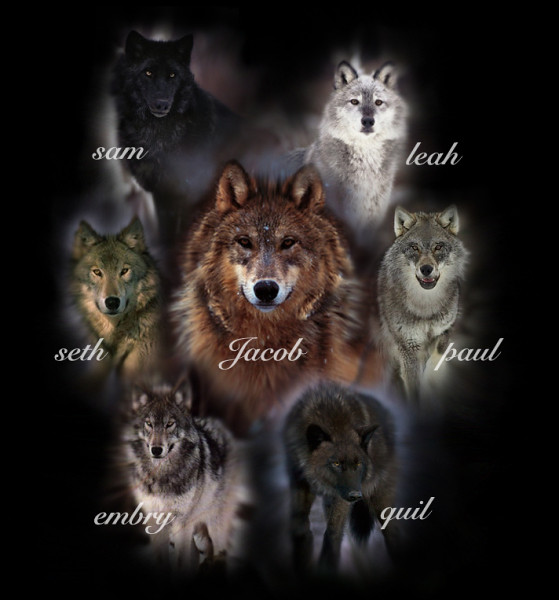The image features a computer-generated graphic of seven wolves, each labeled with a name in cursive white writing against a black background. At the top left is Sam, a black wolf, while the top right shows Leah, a gray, white, and black wolf. Positioned in the middle left is Seth, a brown wolf; at the very center, Jacob, a rust-colored wolf, has the largest picture. To Jacob's right is Paul, a gray and white wolf. On the bottom left, there is Embry, a black, gray, and white wolf, and at the bottom right is Quill, a black and brown wolf. Each wolf's name has only the first letter capitalized, emphasizing the visual hierarchy with Jacob prominently in the center.